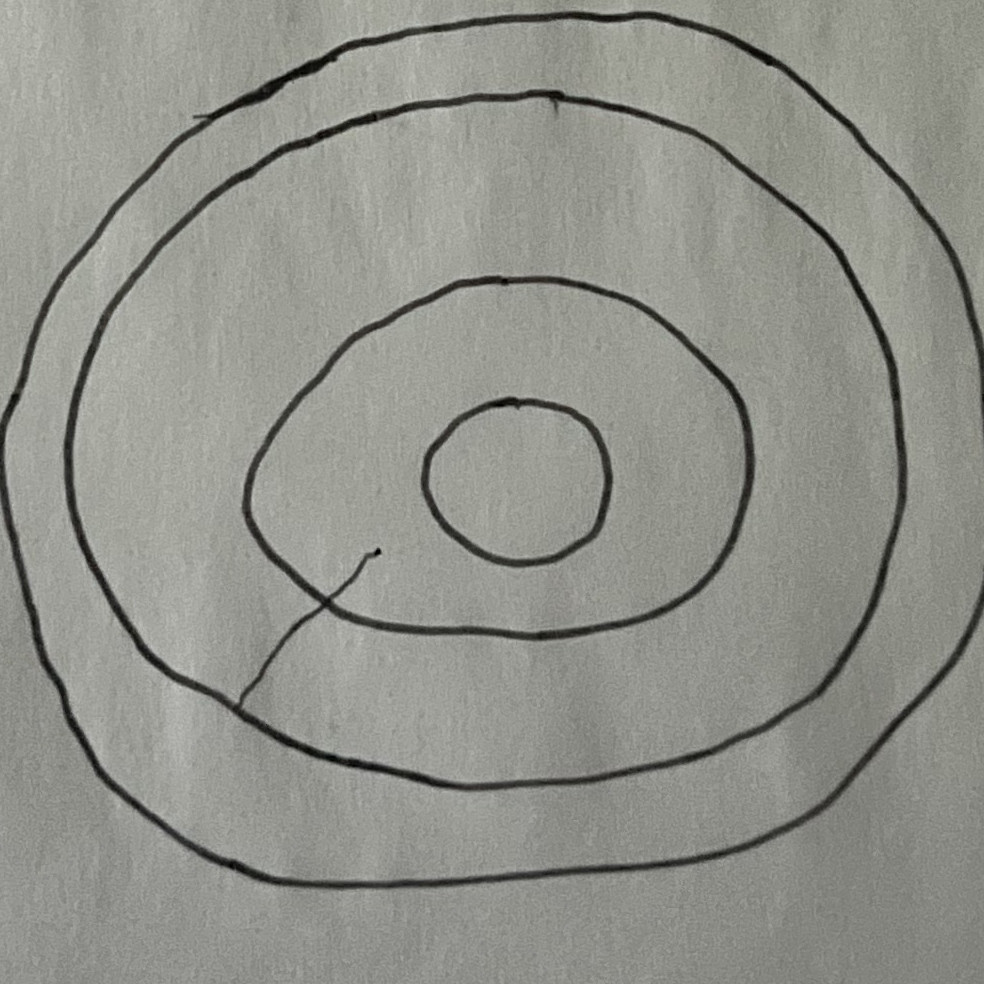This image features a hand-drawn illustration of a target composed of four concentric circles on a textured, neutral gray background. The circles, imperfect and freehand, are drawn in black felt-tip marker, revealing visible overlaps at the points where the lines intersect. The outermost ring encircles three progressively smaller rings, culminating in a central circle.

Additionally, a diagonal line starts from the lower left corner, intersecting the third ring and extending partly into the second ring’s area. This line moves towards the center but does not reach the innermost circle. The entire composition, marked by the raw texture of the paper and the bold black lines without any added colors, creates a stark and minimalistic depiction of a target.